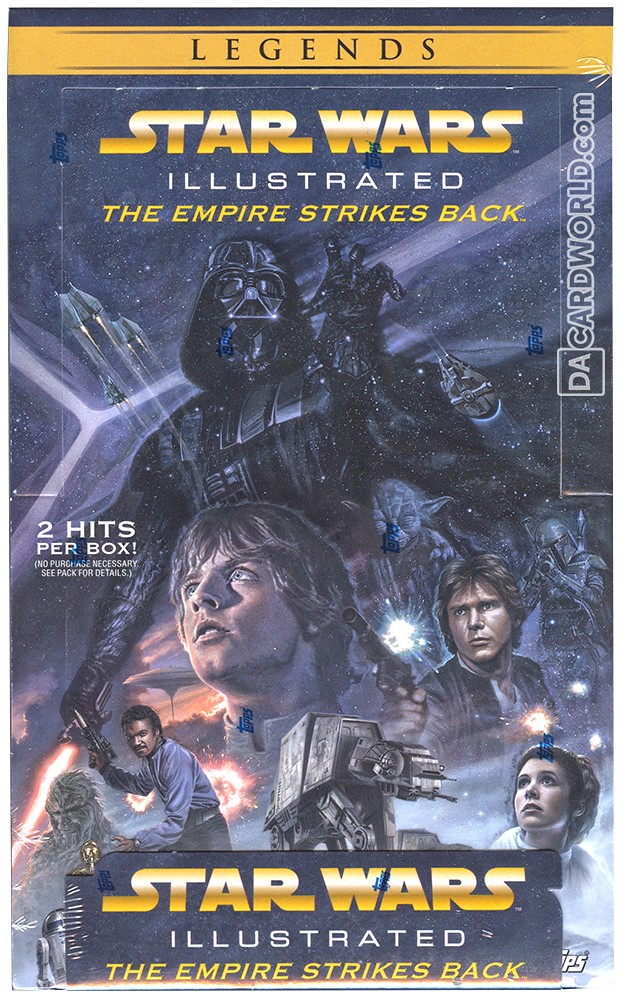This is an image of a sealed box of trading cards for the Star Wars Illustrated series, specifically "The Empire Strikes Back." At the top, a gold bar displays the word "Legends" in black text. Below, in gold and white, is the title "Star Wars Illustrated The Empire Strikes Back." On the right side of the image, "dacardworld.com" is written vertically. The box promises "Two hits per box" and states "No purchase necessary, see pack for details."

The background features a detailed, almost painted scene from the Star Wars universe, with dominant colors of blue, white, black, and gold. Darth Vader looms large in his black uniform at the top of the image, while below him are key characters: Luke Skywalker and Han Solo. Han Solo, positioned to the right and holding a gun, is joined by Princess Leia in the bottom right corner, along with Calrissian, Chewbacca, C-3PO, and Yoda. Boba Fett also makes an appearance. The image includes several iconic ships and elements from the series. At the bottom of the poster, the logo "Star Wars Illustrated The Empire Strikes Back" is repeated, reinforcing the cohesive theme of this vintage-styled collectible.